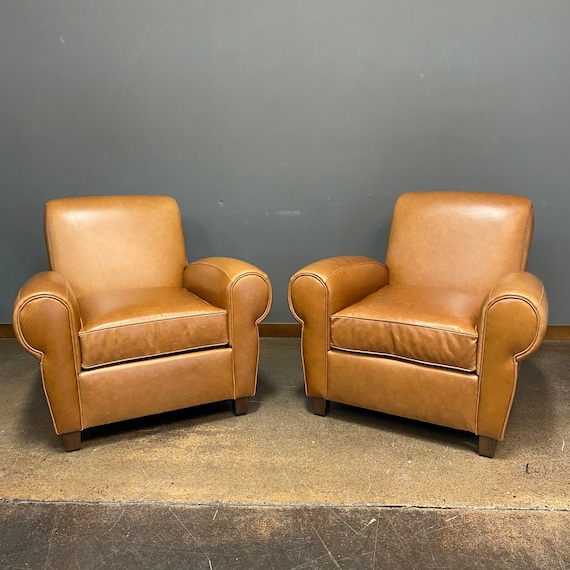This image depicts a pair of slightly worn, light to medium brown leather armchairs, possibly with an orangish or butterscotch hue. The armrests of these chairs are high and arched, featuring a puffy design that tapers down to small, dark wooden pedestal legs. The chairs are relatively wide in the seating area, suggesting ample comfort. Positioned on a gray and brown concrete floor, the chairs face each other slightly, enhancing the composition. The background features a smoke gray painted wall with visible dense marks and scuffs, complemented by a wooden baseboard running along its base. The overall setting conveys a modern and minimalist aesthetic.